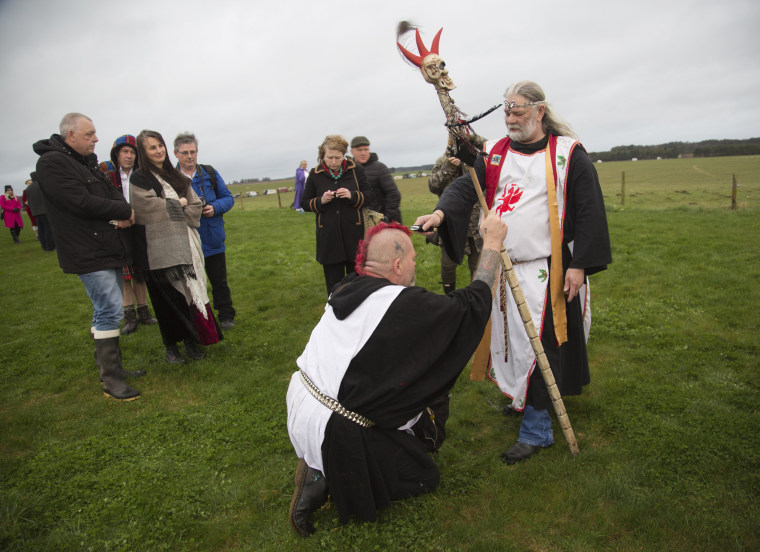In the realism photograph, a medieval-themed event unfolds on a large, grassy field under a gray, overcast sky. In the center of the image, two actors are the focal point, surrounded by a group of onlookers clad in winter coats. The observers, six in total, include a man wearing a black jacket, jeans, and gray boots, and a woman standing in front of him, donning a tan jacket over a possible dress. Another man with a hooded blue and red jacket and another in a black jacket with a backpack watch intently. Nearby, another couple also observes the scene.

The actors are dressed in elaborate costumes reminiscent of monk robes. The standing actor, with long gray hair and a beard, wears a black robe beneath a white cassock adorned with a red dragon emblem and scapulars. He extends a sword towards a kneeling man as if knighting him or bestowing a blessing. The kneeling actor, with a striking red mohawk and a tattoo on the side of his head, wears black and white monk robes and holds a staff topped with a skull featuring its own red mohawk. The intricate details of the actors' costumes and the expressions of the onlookers create a striking contrast between the medieval and modern elements in the scene. The distant treeline and indistinct buildings provide a serene backdrop to the vivid tableau being observed.